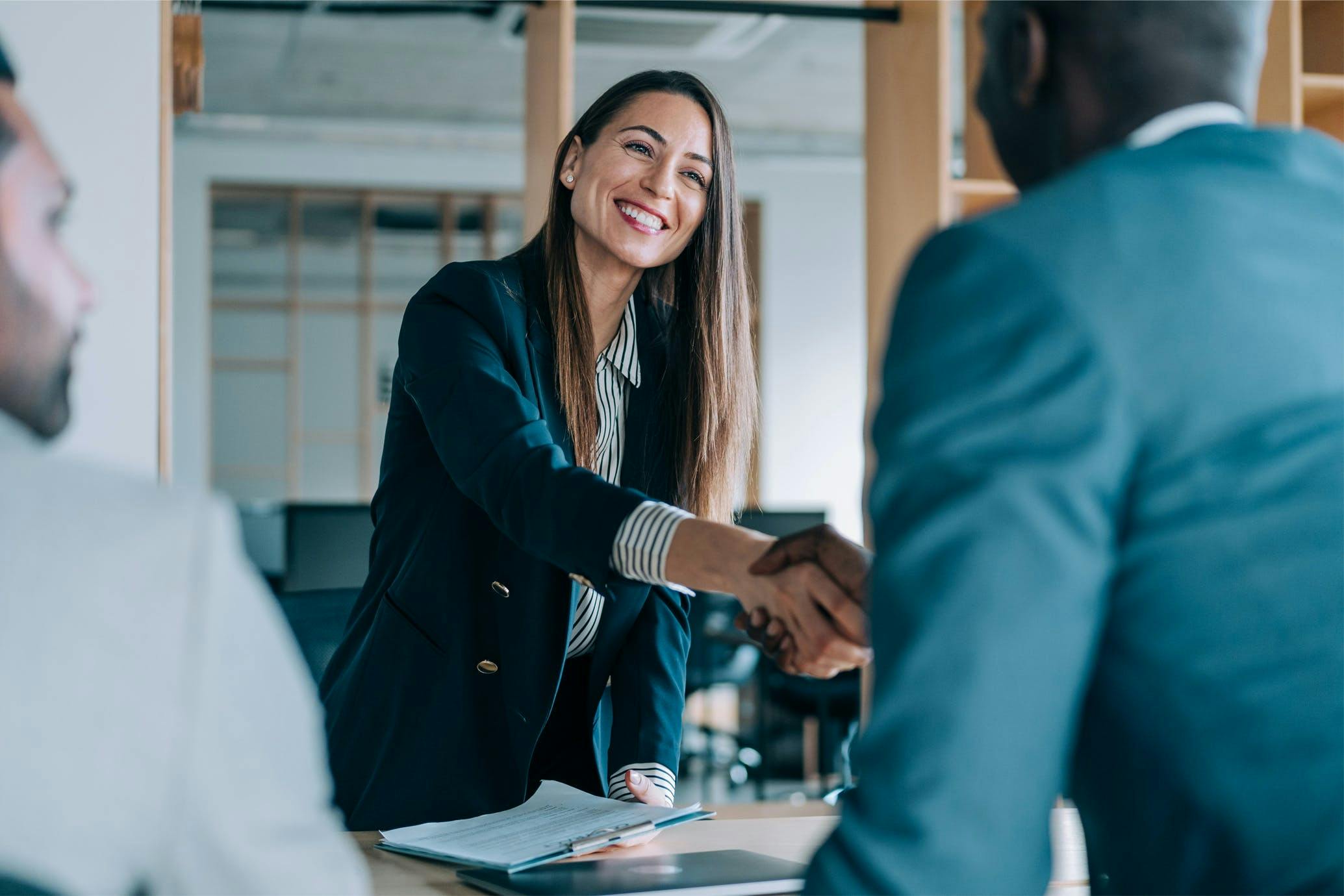In this photograph, a Caucasian woman in her mid-30s with long, straight brown hair and slightly tan skin is shaking hands with an African-American man in a dark blue suit jacket. She is dressed in a striped button-down shirt and a dark blue blazer. She’s smiling broadly, showing her teeth. Beside them is another African-American man sitting down and watching the handshake. He is wearing a light gray jacket. The setting appears to be a business meeting room with white walls and office chairs visible in the background. There is a table with a clipboard and papers on it, suggesting a professional context. The overall atmosphere is one of formality and business.